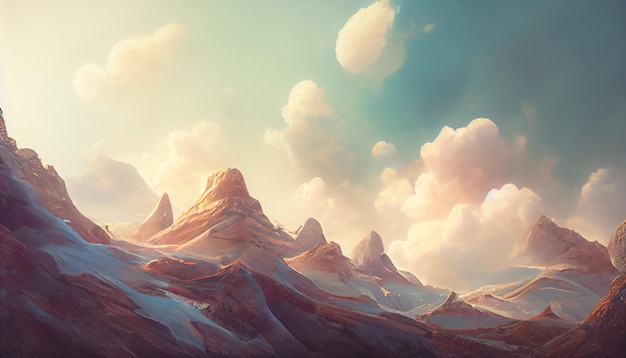The image portrays a fantastical mountain landscape on an alien world. It's a rectangular print, measuring roughly five inches wide and three inches high. The scene features steep, spike-like mountains that dominate the lower half of the image. These mountains exhibit a light reddish-brown color, glowing in the hues of an orange-tinted sky, suggesting the time is either just after sunrise or before sunset. Among the mountains, patches of grayish snow are visible.

At the base, the terrain is darker, gradually transitioning to illuminate the tall, jagged peaks. Rising behind the mountains are thick, fluffy white clouds, radiantly lit by a bright light in the upper left corner, which bathes the clouds in a yellowish glow. The sky above these clouds shifts in color from a light greenish center to a dark greenish-gray blue in the upper right corner, resembling an otherworldly, aqua blue or neon green palette. This ethereal sky further enhances the surreal and fantasy-like atmosphere of the scene. The overall details appear somewhat blurry, characteristic of an AI-generated image or an illustration, further emphasizing its unearthly quality.